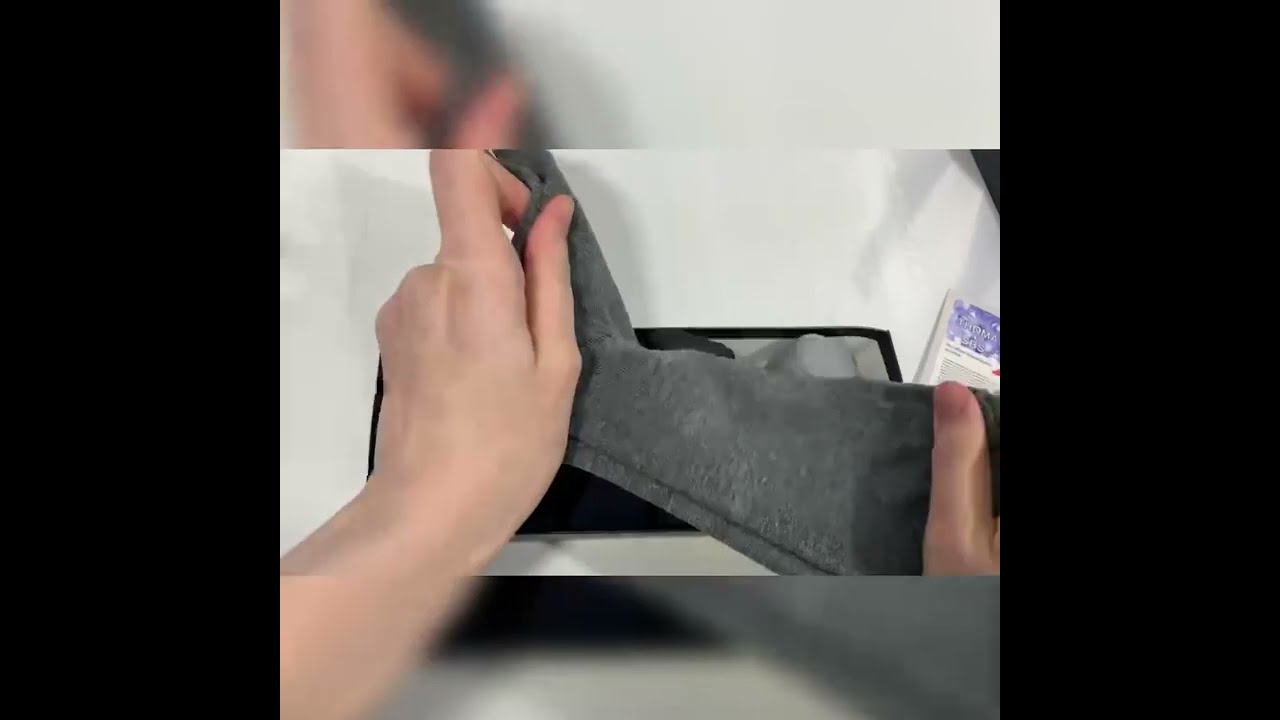The image captures a close-up point of view of someone stretching a gray heather-like fabric with both hands at the center. The left hand, with an index finger bent, and the right hand, with a visible thumb, pull apart the fabric against a white surface. In the background, there is a recessed cubby or doorway rimmed with a black lining. On the right side of the frame, adjacent to the person's right hand, is a tan-colored packet featuring a purple and white label with various small black print. The image is framed by two black rectangles on the left and right sides, enhancing the focus on the central subject. The top and bottom portions of the image are blurred, drawing further emphasis to the horizontally oriented central scene.